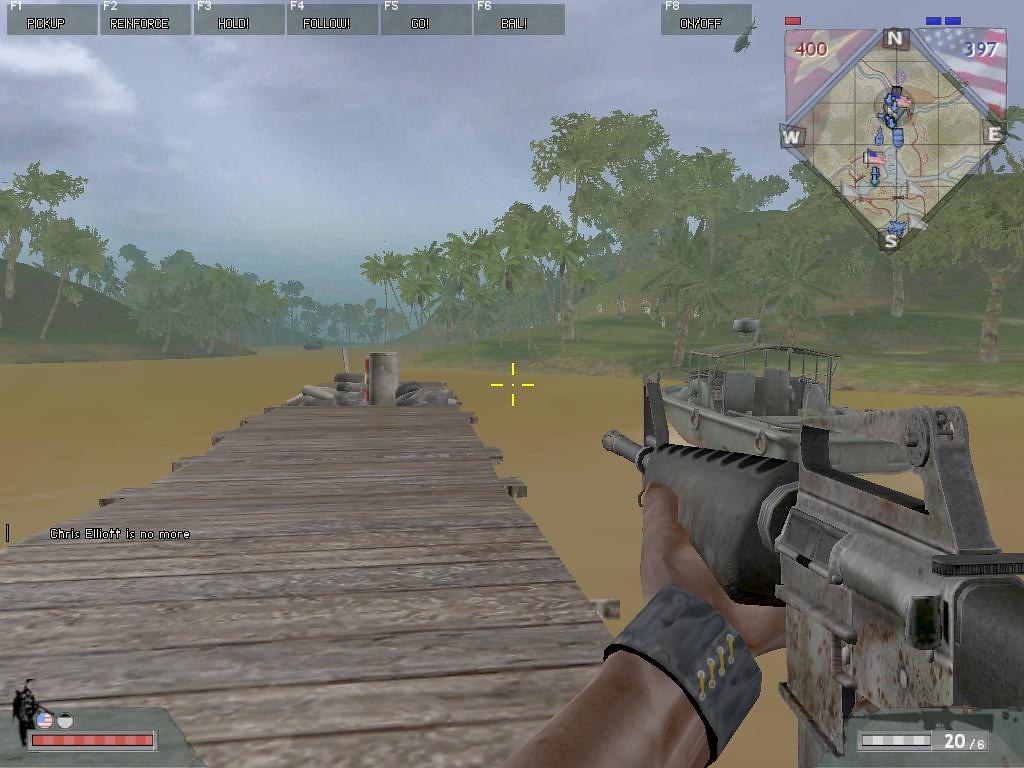In this detailed screenshot from a first-person shooter video game, the central focus is on a player's avatar holding an assault rifle. The rifle's front end and barrel are prominently displayed in black, gripped securely by a hand with a visible portion of an arm adorned with a black leather bracelet. The perspective is through the character's eyes, creating an immersive experience.

Ahead, a wooden dock extends over murky, greenish water, leading towards a background filled with pixelated trees and dense foliage, evoking a sense of wilderness or a remote environment. In the upper right corner, a mini-map is visible, aiding the player in navigation with its green, brown, and black color scheme, reflecting the natural surroundings. The overall visual is dominated by earth tones, emphasizing the game's rugged, outdoor setting.